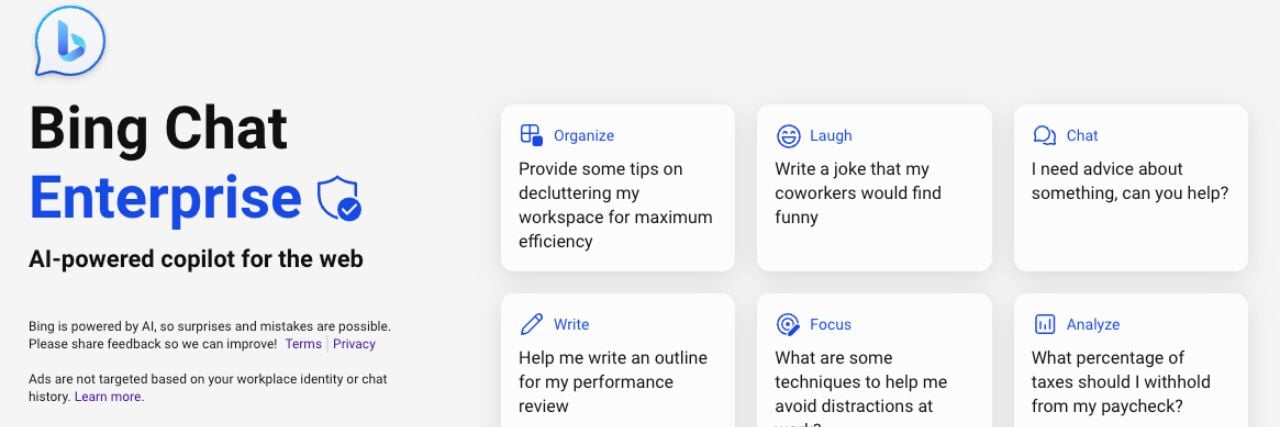The screenshot features a gray background and contains several distinct elements central to its design. 

There is a prominent circle with a check mark, alongside a chat icon and a blue "B," both symbolizing Bing Chat and Black Enterprise, also in blue. This badge is likely indicating an AI-powered copilot for web usage.

Below this are six white squares, each with text and a blue-highlighted command word. They present various features and commands:
1. The first square has the word "Organize" in blue, followed by the text: "Provide some tips on decluttering my workspace for maximum efficiency."
2. The second square features "Laugh" in blue, along with the prompt: "Write a joke that my coworkers would find funny."
3. The third square displays "Chat" in blue, with the phrase: "I need advice about something. Can you help?"
4. The fourth square highlights "Write" in blue, reading: "Help me write an outline for my performance review."
5. The fifth square has "Focus" in blue, with the request: "What are some techniques to help me avoid distractions?"
6. The final square contains "Analyze" in blue, but the text is partially cut off, starting with: "What percentage of taxes should I withhold from my paycheck?"

This detailed depiction illustrates the use of an AI tool designed to assist with various tasks, efficiently organized through interactive and intuitive options.